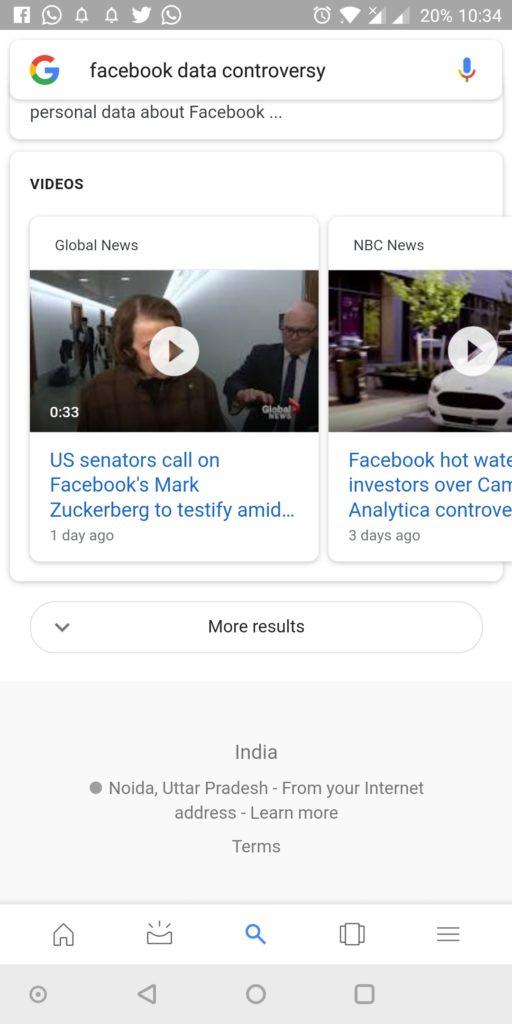The image captures a screenshot taken on an Android smartphone, evident from the status bar at the top of the screen. The user has searched for "Facebook data controversy" on Google. The search results showcased include two video thumbnails: one from Global News and another from NBC News. 

The Global News video is 33 seconds long and is titled "U.S. Senators call on Facebook's Mark Zuckerberg to testify amid...," posted one day ago. The NBC News video title is partially visible, reading "Facebook and Hot Water investors over...," and was posted three days ago. There's an option to view "More Results."

The footer of the screenshot displays the search toolbar, with icons for Homepage, News, Video, Menu, and Search functions. The time on the device shows 10:34, without indication if it’s AM or PM. The status bar indicates multiple notifications from apps like Facebook, WhatsApp, and Twitter, among others. The geo-location note mentions "India, Noida, Uttar Pradesh" based on the user's internet address.